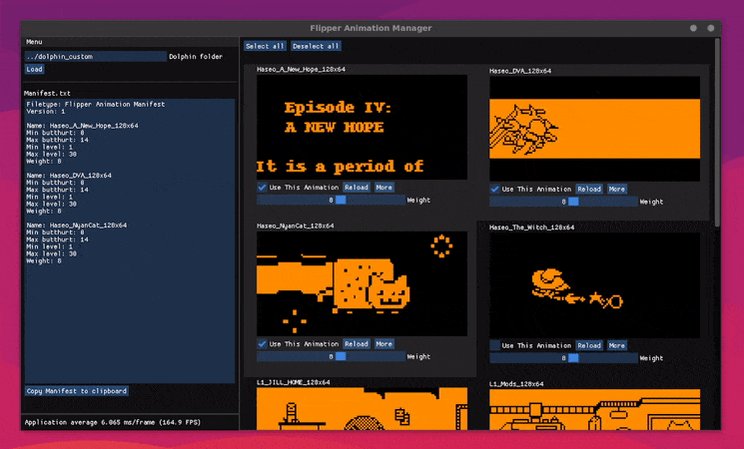This image showcases a computer interface titled "Flipper Animation Manager" with a prominent pink and purple border. In the upper center, the phrase "Flipper Animation Manager" stands out, while the page is divided into multiple sections and digital windows. On the left side, there is what appears to be a code management area divided into three sections, featuring various lines of code in white text on a gray background. Below this, a line reads, "Copy manifest to clipboard," followed by another line stating, "Application average 6.065 me frame."

The main interface is horizontally rectangular and divided into several smaller, orange-tinted windows. In the top left section, the text reads "Episode 4, A New Hope. It is a period of," suggesting a reference to "Star Wars." Adjacent to this window, on the right, is another orange panel containing some form of black text or design that is difficult to discern. In the left center window, there is an image resembling Nyan Cat, while the right center image depicts a scene with a cowboy hat and a figure reaching out to touch a star. Toward the bottom, partially cut-off and less distinguishable, there are more images including one with orange hues and another potentially depicting a witch character. Overall, the detailed and multi-colored imagery combined with the coding elements suggests a dynamic tool for managing and animating various digital assets.